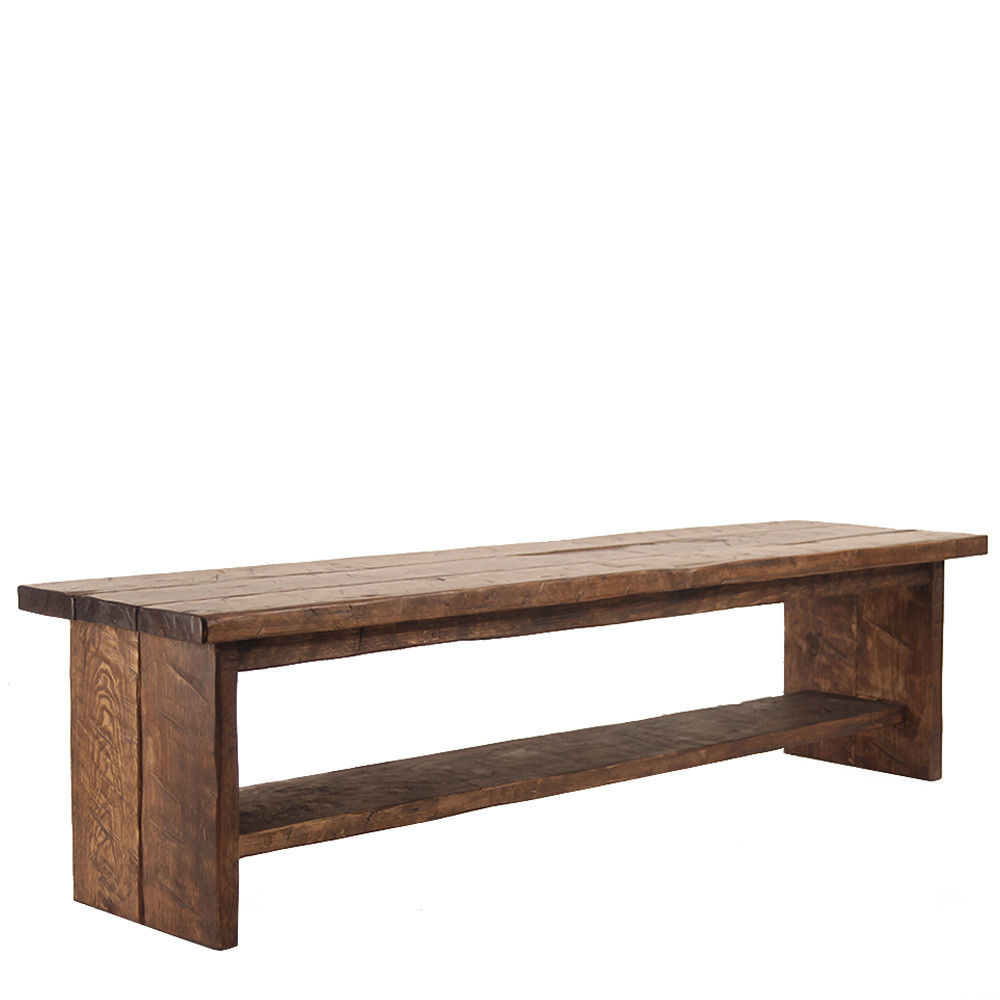This color photograph features a long, narrow wooden bench against a white background, highlighting its sturdy, well-constructed design. The bench's top is composed of three long planks of dark brown wood that have been stained and sealed with a shiny finish, possibly a deep mahogany tone. Supporting the top are two rectangular wooden legs, each made from two-by-fours, and connected by a single wider beam running horizontally for added stability. The visible wood grain and fine quality of the wood suggest careful craftsmanship, giving it a primitive yet refined appearance reminiscent of furniture from the Amish country. The bench's clean lines and solid construction make it versatile enough to be used as a shelf or a table in various settings such as an office or dining room.